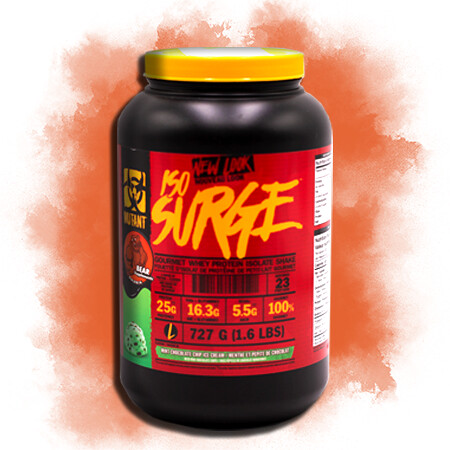This image depicts a low-resolution bottle of protein powder designed for weightlifting enthusiasts. The bottle is black with a bright yellow cap and prominently features a striking red label. The product name, "ISO Surge," is emblazoned across the label in a chaotic, graffiti-like yellow font. The main branding "150 Surge" has a small '150' and an exaggerated 'Surge,' with the middle letters enlarged and the 'E' jutting out. The overall design style is reminiscent of 90s radicalism, conveying an edgy and cool aesthetic.

Below the main title, the label mentions "gourmet whey protein isolate shake" in a mix of yellow and blue text. Additional details are harder to discern due to the image's resolution. To the left side of the label, there is a flash of green that appears to depict a scoop of mint chocolate chip ice cream, hinting at the flavor. A yellow square near the top features a biohazard symbol and the word "Mutant," reinforcing the hardcore branding. On the right side, a section of the label is white, likely containing the nutritional information. The entire package weighs 1.6 pounds, as mentioned on the label.